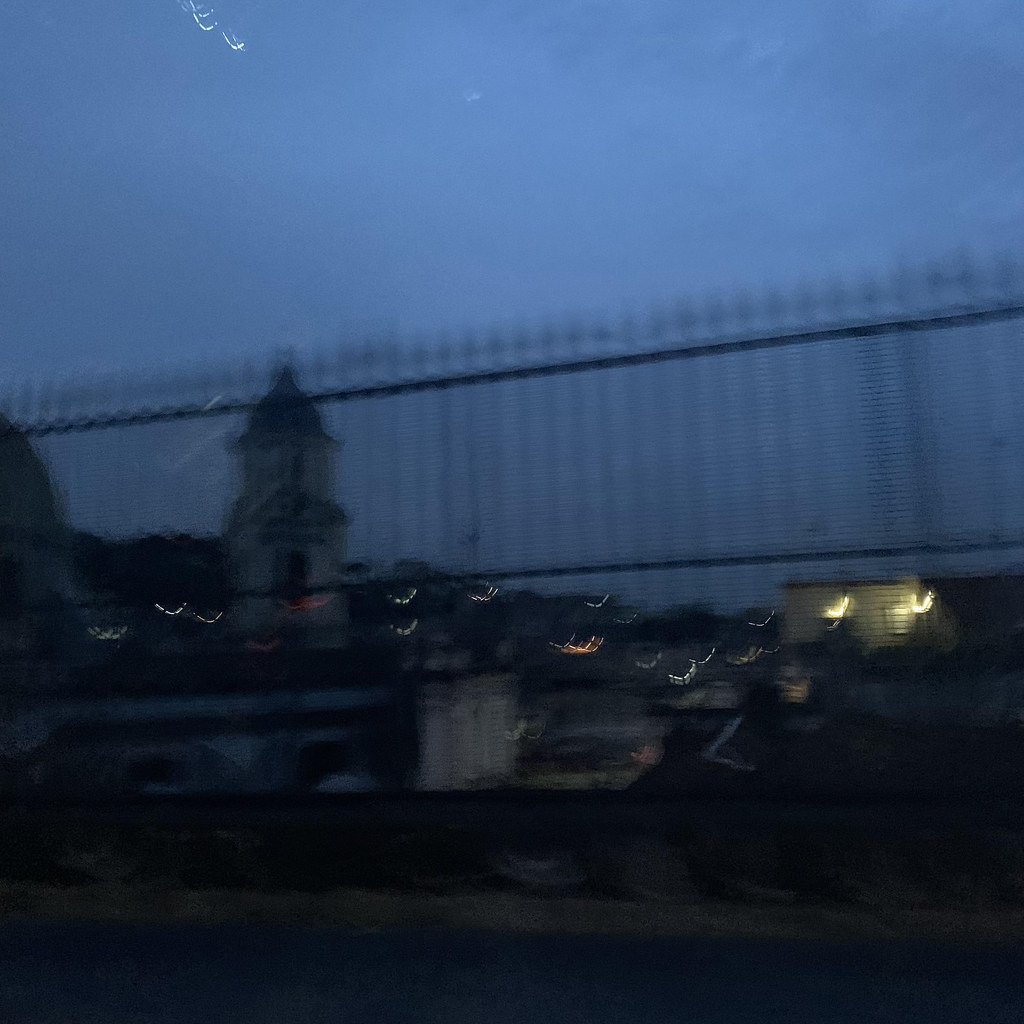This nighttime cityscape photograph features a dark blue sky and is notably blurry, suggesting it was taken in motion. On the right side of the image, there's a one-story building that could be interpreted as a house or a shop, possibly in a tan or white color. On the left side, a larger structure that resembles a church dominates the scene. This slender, rectangular building is capped with a distinctive dome that flares out at the sides, appearing quite dark in the photo. In the foreground, a black metal fence with arrow-shaped points and numerous vertical bars frames the scene, adding to the urban atmosphere of the composition.